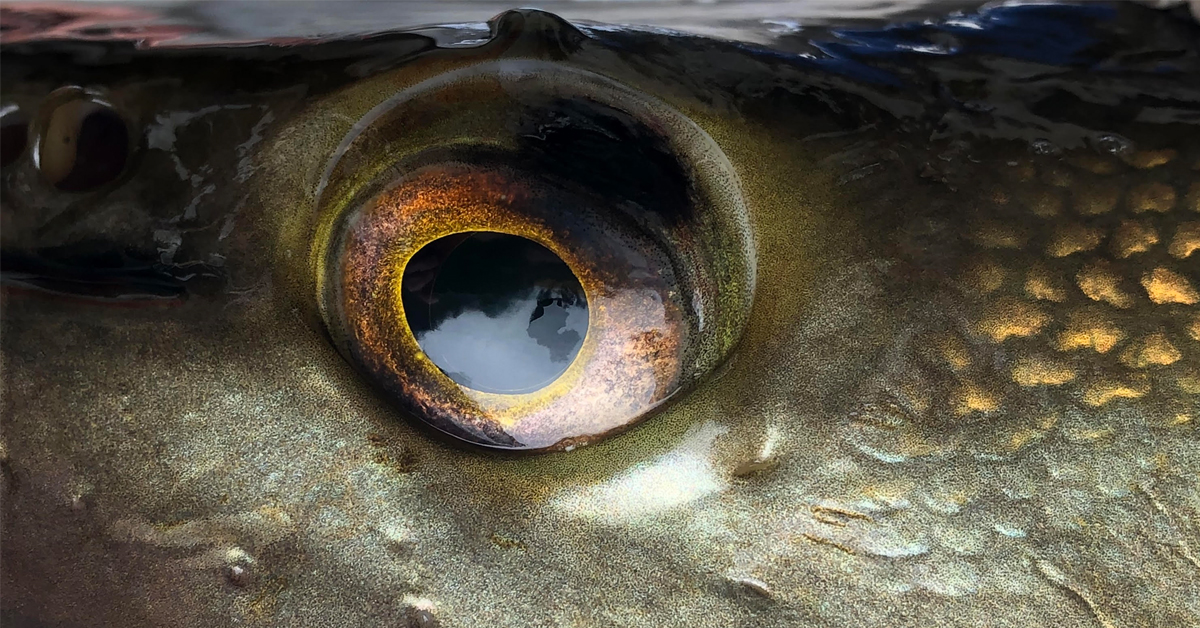This close-up image showcases the eye of a mysterious creature, possibly a fish, frog, or even a dragon-like figure, emphasizing its smooth, scaly, bronze-gold face. The shimmering, reflective scales glow in hues of gold, bronze, and yellow, while the eye itself commands attention at the center of the image. This large, wet-looking eye is surrounded by deep orange and yellow tones, leading into a strikingly deep black pupil, speckled with hints of yellow and orange. The artistic style of the image highlights the magnified details of the scales and the eye, giving it a jelly-like texture that shimmers and glows under the light. The overall color palette melds golden bronze with splashes of brown, black, orange, and green, creating a visually captivating and enigmatic portrait.